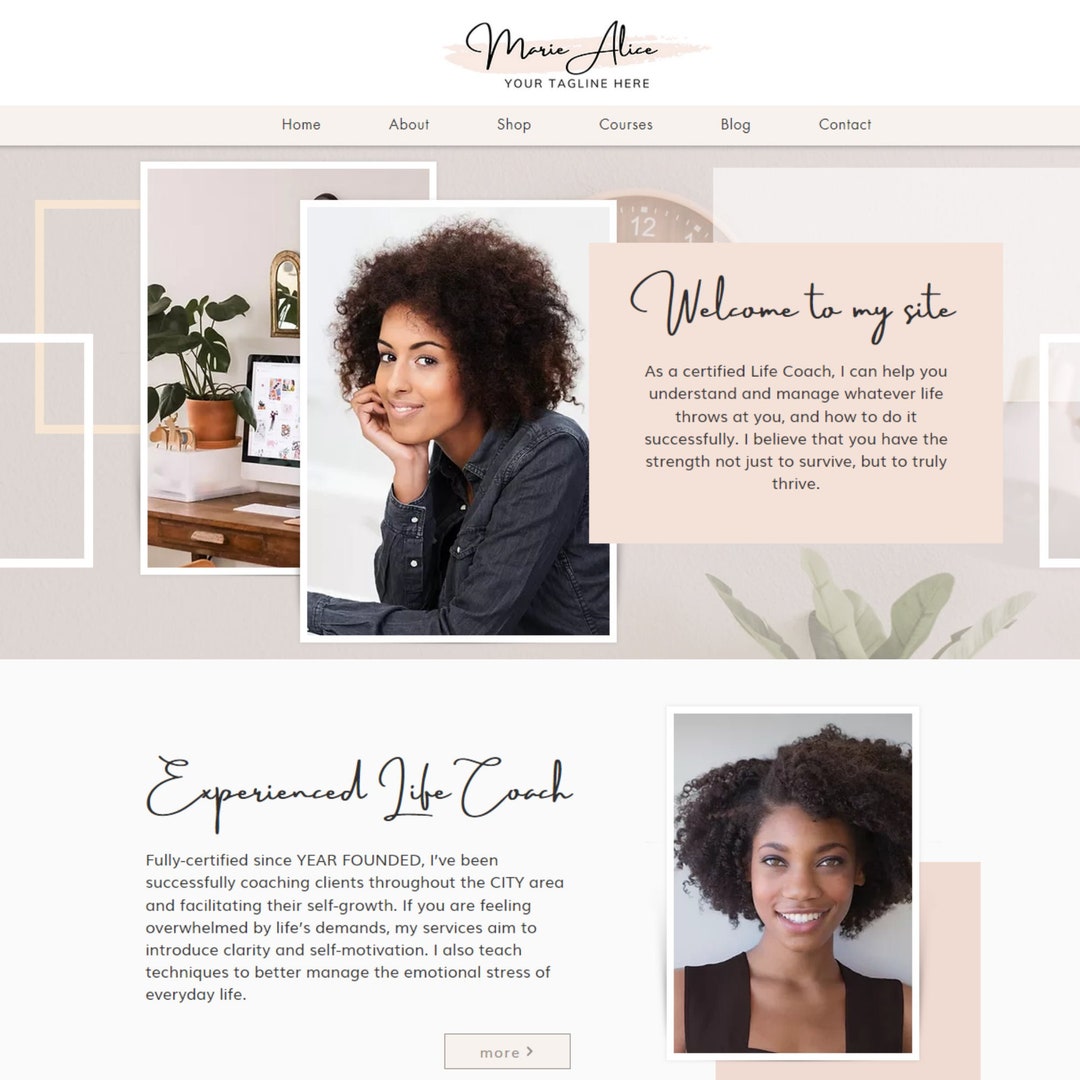Homepage of Marie Alice, Certified Life Coach

At the top of the website's homepage, "Marie Alice" is prominently displayed in elegant fonts, creating a warm and inviting introduction to her digital space. Just beneath her name sits a placeholder for her tagline, waiting to encapsulate her mission and vision in a concise phrase.

The navigation bar sits snugly within a subtle tan border, offering seamless access to various sections of the site: Home, About, Shop, Courses, Blog, and Contact. These links guide visitors effortlessly through Marie's comprehensive offerings.

Dominating the top portion of the page is an image capturing her meticulously curated office space. In this snapshot, viewers see a sleek desk adorned with a computer monitor and a vibrant green plant, infusing the space with life. Personal touches in the form of framed pictures hang on the wall, imparting a sense of warmth and individuality.

To the right of this setup is a striking photograph of Marie Alice herself. She appears to be a biracial woman with a head full of luscious, curly hair. The photo captures her in a reflective pose, with her chin resting thoughtfully on her palm. She exudes a calm, approachable demeanor, dressed casually in a long-sleeve denim shirt reminiscent of a Wrangler dungaree.

Beneath her photograph, a welcoming message invites visitors deeper into her world: "Welcome to my site. As a certified life coach, I can help you understand and manage whatever life throws at you and how to do it successfully. I believe that you have the strength not just to survive, but to truly thrive."

Further down the page, more details about her professional credentials and experiences are displayed: "Experienced Life Coach, Fully Certified Since [Year Founded]. I've been successfully coaching clients throughout the city area and facilitating their self-growth. If you are feeling overwhelmed by life's demands, my services aim to introduce clarity and self-motivation. I also teach techniques to better manage the emotional stress of everyday life." A “More” button invites users to explore further details of her journey and testimonials.

The homepage concludes with another photograph of Marie Alice, reinforcing the connection between the coach and her potential clients, and adding a personal touch to the professional atmosphere of the site.